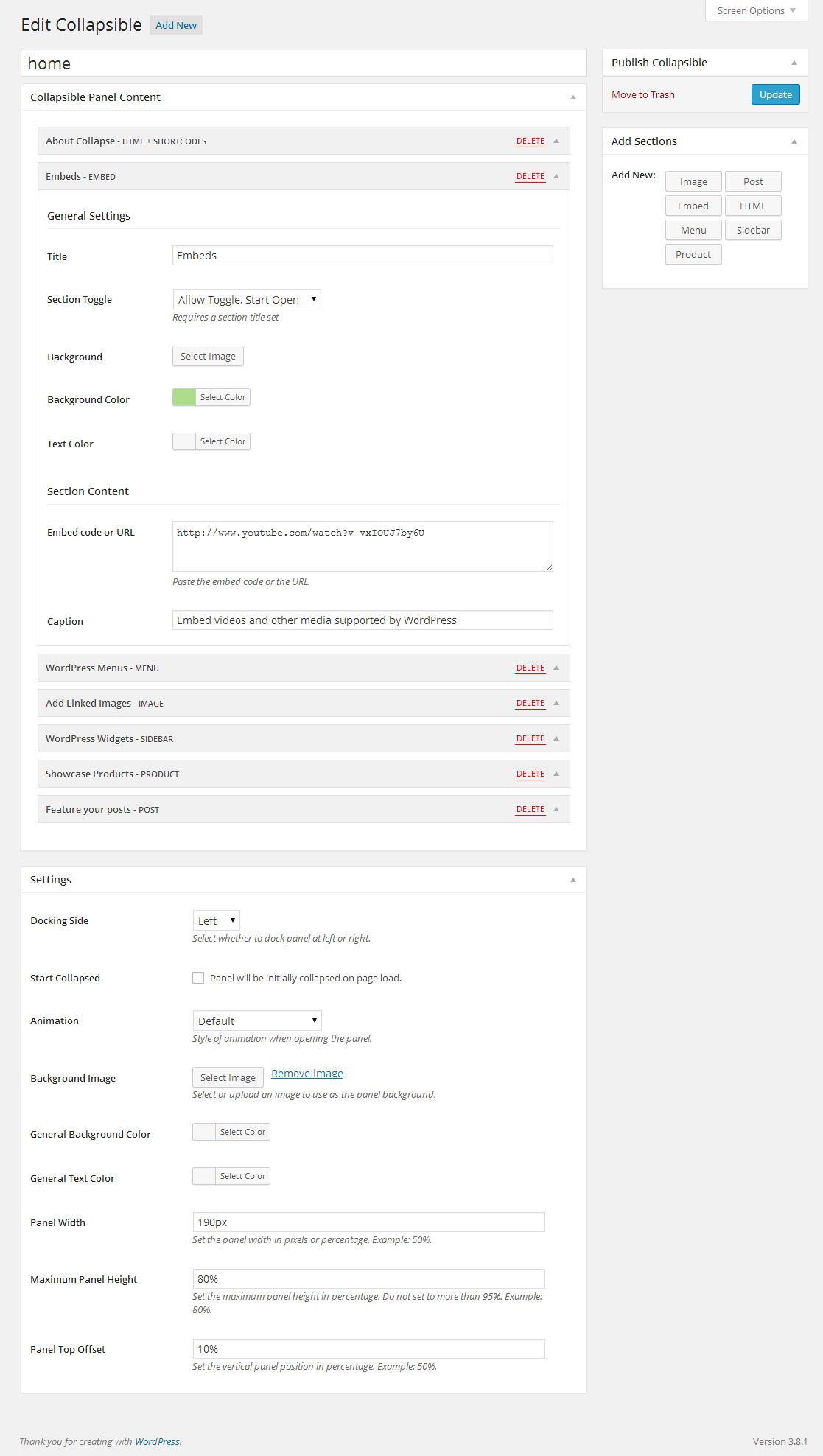In the image, a user interface is displayed with a focus on configuring collapsible sections, presumably for a website or application. The background is a visually muted gray, with multiple white columns containing text and settings options.

**Top Section:**
- The **top left-hand corner** features the label "Edit Collapsible," accompanied by a button labeled "Add New."
- The **top right-hand corner** contains a link to "Screen Options."

**Left-Hand Main Column:**
- The first visible section under "Edit Collapsible" is labeled "Home."
- Within this primary column, there's a subsection titled "Collapsible Panel Content" that offers tabs or options related to collapsible elements, embeds, and general settings.

**Settings Configurations:**
- Users can assign a title to a section with a "Section Toggle."
- There are options to select a background image and choose a background color.
- Text color can also be selected.
- For "Section Content," users are allowed to embed code or URLs. In this instance, "www.youtube.com" has been inputted.

**Additional Options:**
- Users can insert captions and configure settings related to the WordPress menu, linked images, WordPress widgets, showcasing products, and featuring posts.

**Bottom Settings Panel:**
- Various settings are available, such as:
  - Choosing the alignment of the document side (left or right), with the left option currently selected.
  - Options for "Start Collapsed" and "Animation Default."
  - Parameters to select a background image, background color, text color, panel width, panel height, and top panel offset.

The interface presents a variety of customization options, providing ample flexibility for users to tailor their collapsible sections according to their preferences or project requirements.